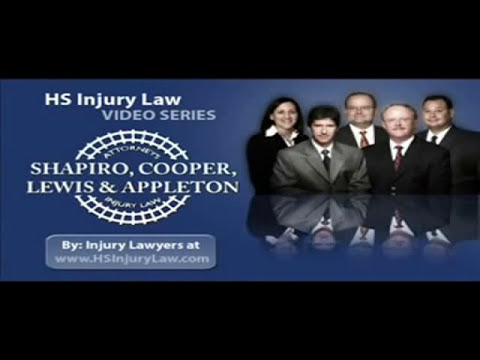This image is a color photograph capturing a still from a video advertisement for the injury law firm Shapiro, Cooper, Lewis, and Appleton. The composition features five attorneys—one woman and four men—standing in professional attire, with their reflections visible on the glossy surface of a table in front of them. On the left side of the image, white text on a blue background announces the "HS Injury Law Video Series," coupled with a circular logo that bears the names Shapiro, Cooper, Lewis, and Appleton. Below this, a gray box reads, "By Injury Lawyers at www.hsinjurylaw.com," informing viewers of where to find more resources. The background is styled with clouds, adding a dynamic element to the setting, and thick black bars frame the top and bottom of the image for emphasis. This advertisement aims to educate and guide individuals on their rights and potential claims related to workplace injuries, ensuring they get the best possible advice and outcome.